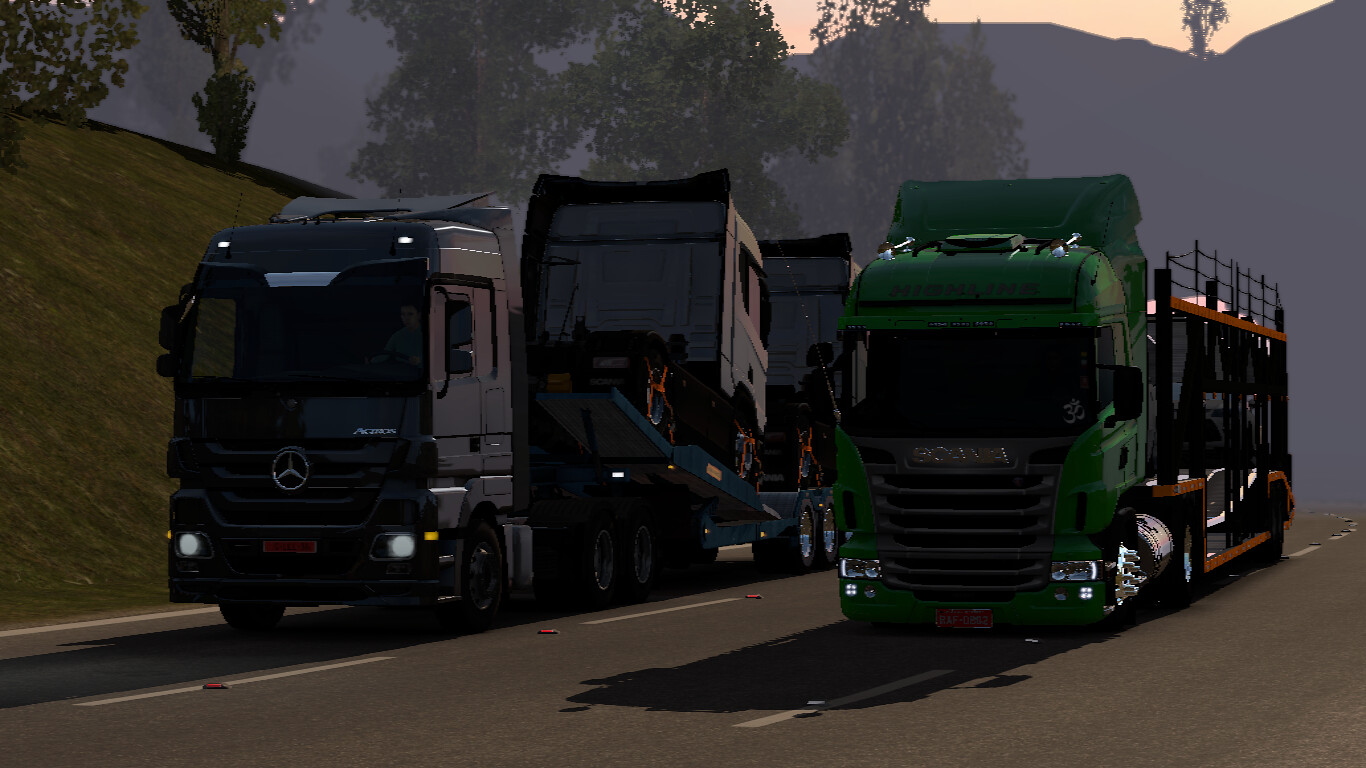In the low-light photograph, two 18-wheelers are depicted driving side by side on a three-lane highway, set against a backdrop of towering mountains dotted with trees. The truck on the left, a sleek and contemporary black Mercedes cab, features headlights illuminating the dim scene. It is hauling several gray cabs adorned with distinctive red rims, secured to a flatbed trailer. In contrast, the truck on the right sports a dark green cab with a decal on its windshield, and it carries a double-deck trailer designed for vehicle transport, devoid of any cars at the moment. The hill beside the road is covered in grass and trees, blending into the expansive, mountainous landscape.